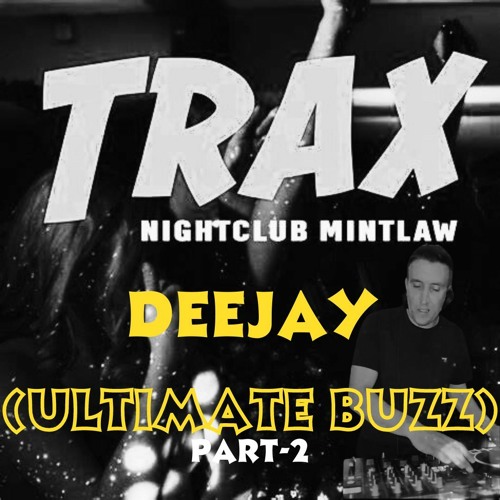The image appears to be a CD cover or an advertisement for a DJ event. Dominating the top section is large white text that reads "T-Rex." Below it, smaller white letters spell out "Night Club Mint Law." A slightly larger yellow text spells out "DJ" as "D-E-E-J-A-Y." Underneath this, the hollow yellow text reads "Ultimate Buzz," followed by "Part 2" in white beneath it. The background, rendered in black and white, features a DJ actively spinning in the bottom right corner. He's interacting with a turntable and a mixing panel replete with multiple knobs and switches.